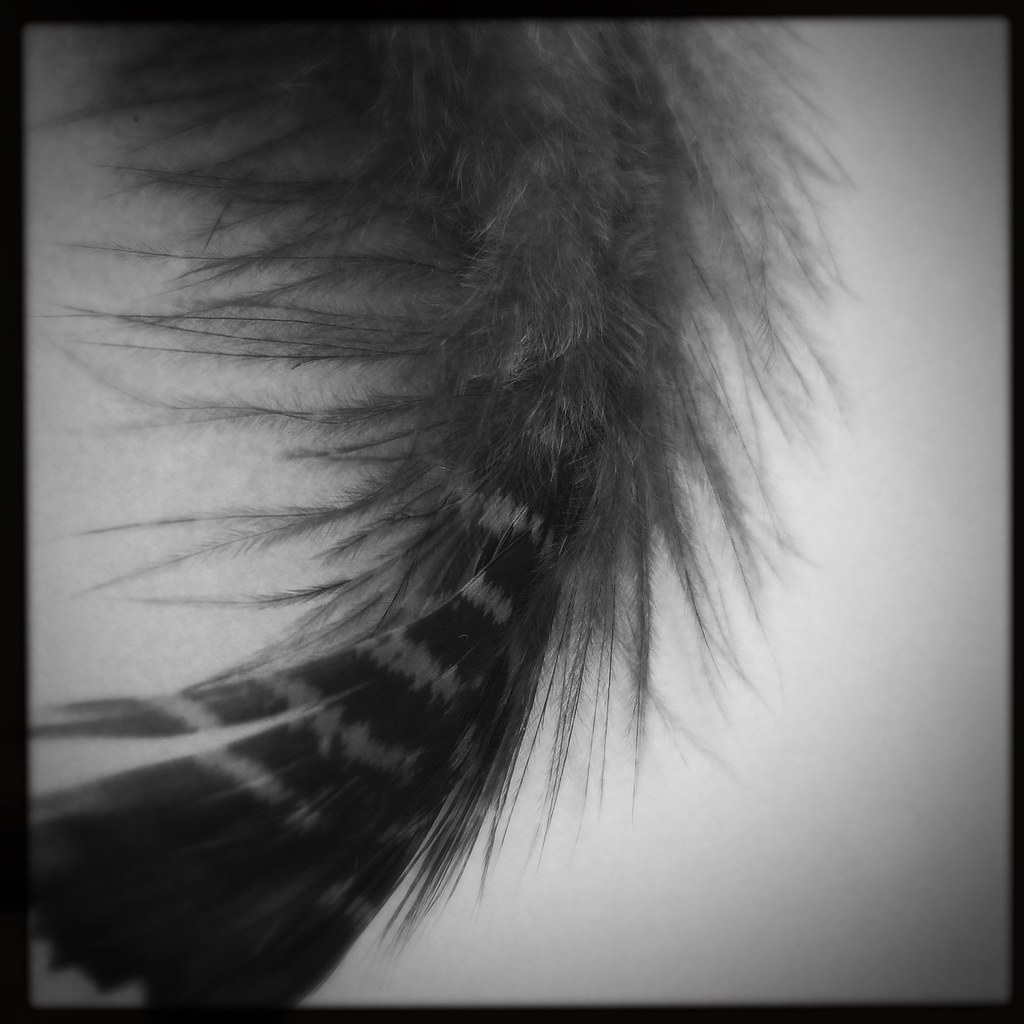This black-and-white photograph presents a close-up of a feather with exquisite detail, emphasizing its soft, intricate structure. The feather, possibly from a turkey, dominates the image as it extends from the bottom left corner and curves gracefully to the left, continuing beyond the top edge of the square frame. The background is a nondescript white surface, perhaps a wall or countertop, subtly blurred to keep the viewer's attention on the feather itself. A thin black border encapsulates the entire image, enhancing its sharpness and framing.

At the feather's lower end, distinct black and white stripes are visible: the tip is all black, followed by alternating thin gray and black stripes. The feather exhibits a smooth and natural appearance here. As the eye travels upward, the feather starts to appear more frayed and wispy, with numerous thinner filaments branching off to the sides, giving it a slightly ruffled and fuzzy texture. This fraying suggests the feather may have seen some wear or could be part of the softer down feathers. The photograph meticulously captures the delicate and graceful details of each tiny strand, underscoring the intricate beauty of the feather in a monochromatic palette.